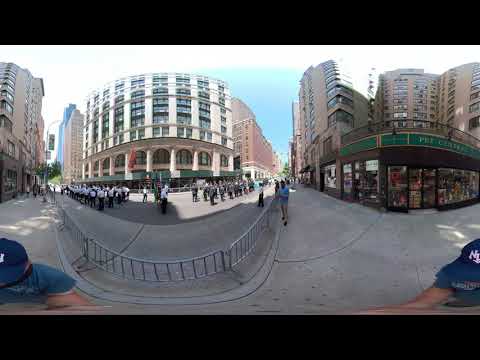This image captures a bustling city scene using a wide-angle or fisheye lens, which distorts the view, curving lines that are actually straight. In the foreground, a person wearing a blue New York Yankees baseball cap and a short-sleeved blue shirt is prominently featured twice, due to the panoramic nature of the shot, with halves of him appearing on both the lower left and right corners. The sidewalk on which he stands is partly enclosed by a curved fence, and behind him, a lively street corner unfolds.

In the midground, there's a parade with two distinct groups of people marching in formation, one dressed in white and black and the other in light gray, all bathed in sunlight. High-rise buildings and about ten-story apartment buildings stretch skyward, creating a bustling urban backdrop. On the right side of the image, a brown storefront with a green banner and glass windows is visible. The store appears to have various indistinguishable objects inside, while the sidewalk bends around the scene, contributing to the expansive city block view.

Most of the people, grouped densely in the background, seem to be participating in or watching the parade, organized neatly into rows and columns. The sky peeks through as a sliver of blue with a touch of white haze at the top of the image, framed by black borders above and below. It's a bright, sunny day, and the shadows of the buildings fall upon the milling crowd, adding depth and vitality to this vibrant cityscape.